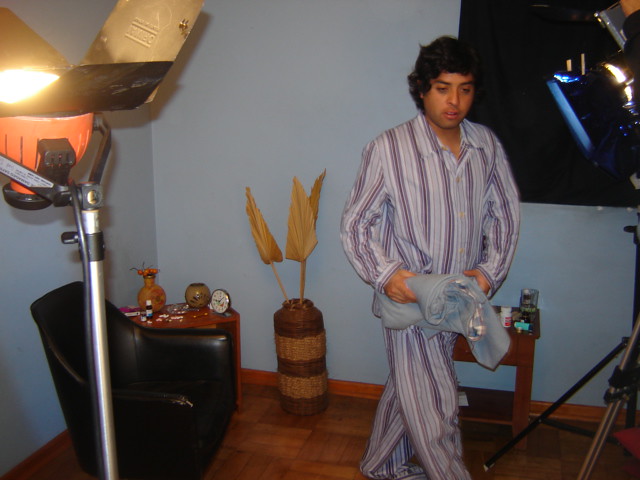This detailed image captures a possibly South Asian man with a brown complexion and wavy black hair, wearing striped pajamas with a white base and navy stripes. He stands, carrying a soft wool blanket or throw in his arms, exhibiting a dazed expression while looking towards the floor and off-camera. His legs are crossed, adding to his contemplative demeanor. The setting appears to be a living room that has elements suggesting a photo studio, such as two large movie-like lights. 

In the bottom left corner, there's a black armchair partially concealing a small wooden side table adorned with various knickknacks, clocks, and jars. A standing photo lamp is also present in the foreground on the left. Additionally, a wicker vase with beige fronds decorates the space. The walls of the room are painted a bluish-gray, adding a neutral but cozy ambiance to the scene.